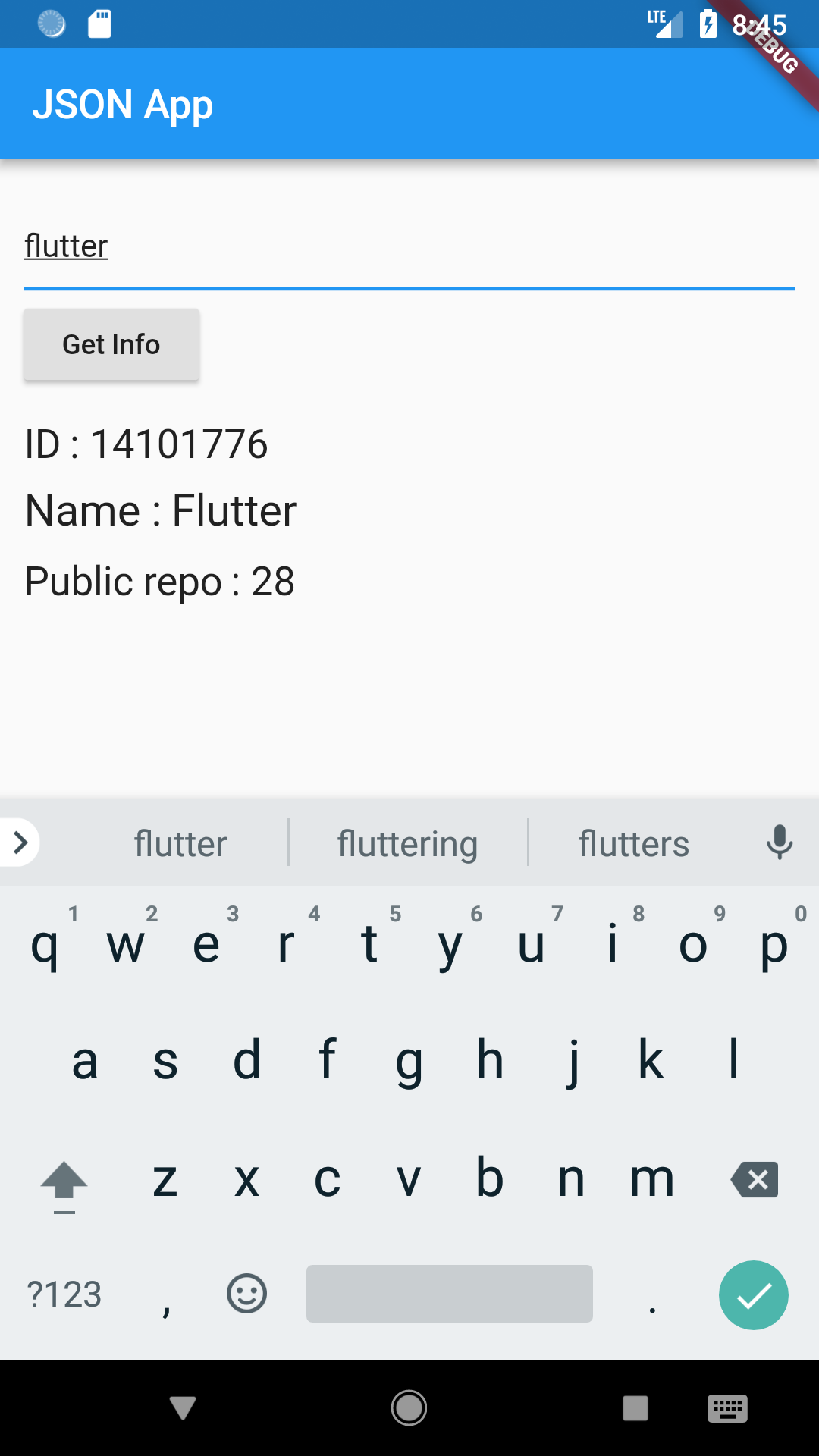This image depicts an Android interface showcasing a JSON-related application. In the upper left-hand corner, the status bar displays the time, battery life, and cellular signal strength. Notably, there is a horizontal red line with white text that reads "DEBUG" situated just below the time on the system UI header.

The app's header prominently features the title "JSON App". Below this title, there is a text box with the word "Flutter" in black, underlined text. Immediately beneath the text box, a gray button with black text is visible.

Further down, three lines of text provide specific details: "ID 14101776", "Name: Flutter Public Repo 28". At the bottom of the screen, the Android system keyboard is displayed, showing three auto-correct suggestions: "flutter," "fluttering," and "flutters," in gray text on a light gray background. There is also a microphone icon to facilitate voice input.

The QWERTY keyboard layout is visible for typing, with keys in black text, a green checkmark icon, and a gray spacebar. At the very bottom, the standard Android system navigation bar is present, featuring icons for back navigation and other options.